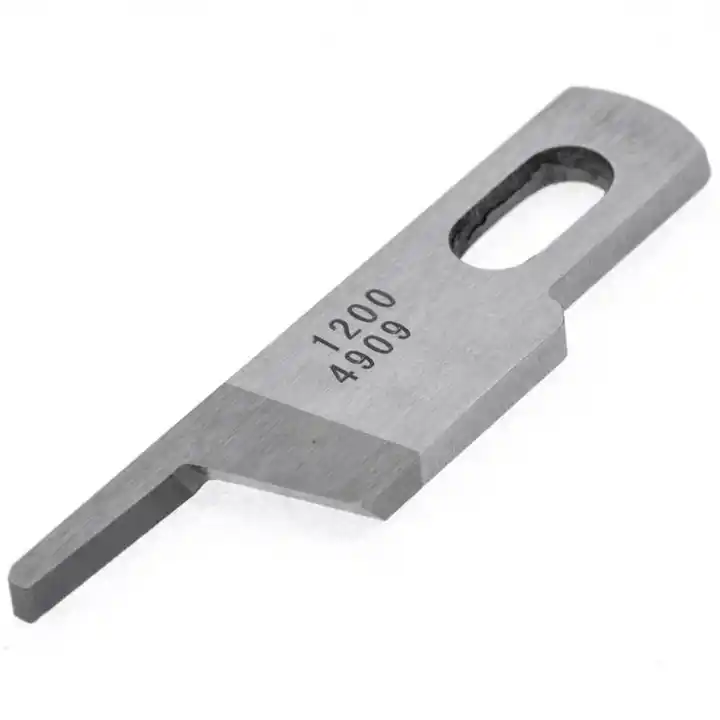The photograph showcases a close-up of a uniquely shaped metal tool set against a pure white background, suggesting a product photo. The tool, angled at 45 degrees from the bottom left to the top right, features a light metallic gray color with a brushed texture. The lower left portion of the tool is slightly darker and tapers into a small protrusion or nubbin. The central and right side of the tool is predominantly rectangular with a rounded end, and contains a semi-circular slot or pill-shaped hole with a rough metal interior. Engraved on the top part of the implement are the numbers "1200" and "4909".